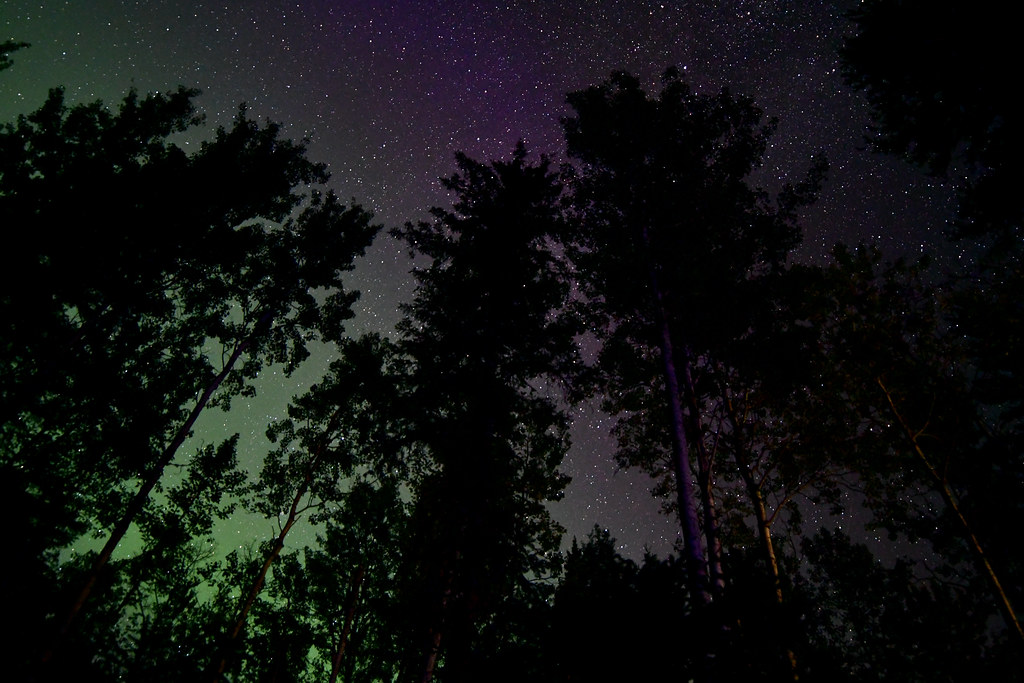This is an evocative, highly-filtered photograph capturing the night sky through the eyes of someone standing in a dark forest. The image is horizontally composed and depicts the silhouettes of towering tree trunks and dense leaves, all outlined in a pitch-black hue. The trees lean slightly inward, enhancing the immersive, upward gaze into the celestial canvas above. The sky itself showcases a mesmerizing gradient: a bright greenish hue dominates the left side, transitioning seamlessly into various shades of royal purple before deepening into a midnight black in the top right corner. Scattered across this vibrant palette are numerous white dots, representing dozens, if not hundreds, of twinkling stars. A golden tint on some tree trunks subtly contrasts the predominant purples and greens, further adding to the ethereal quality of this night sky scene.